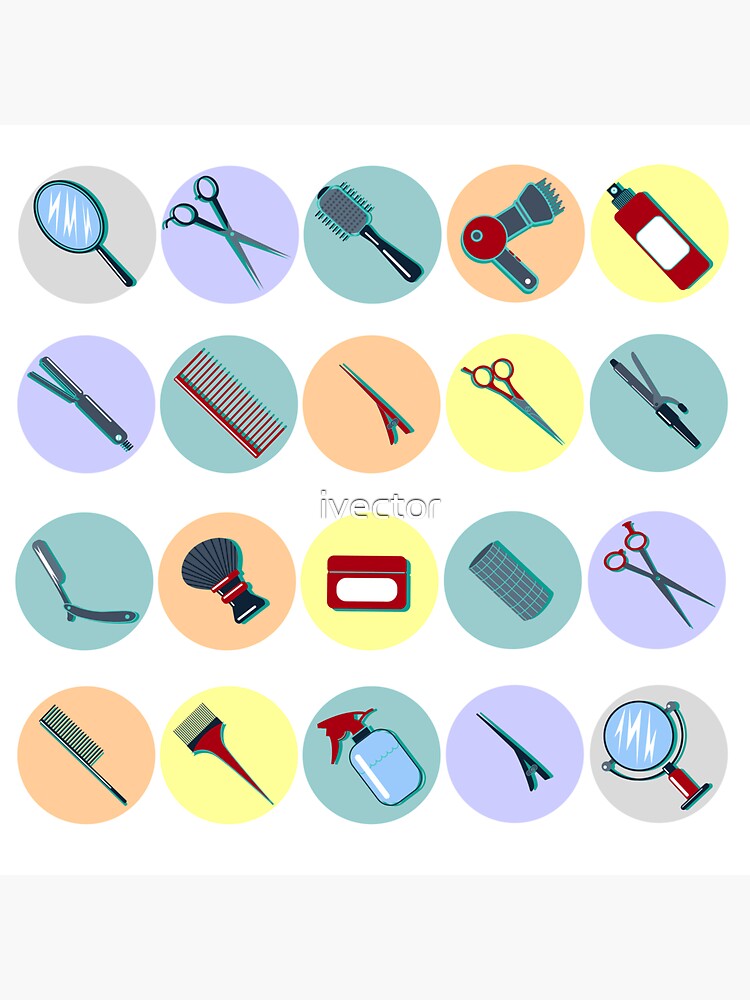The image is a detailed layout featuring a multitude of colorful circles, each containing distinct cosmetology and hairdressing items. The circles are arranged against a white background in a square pattern, with a bold "I-VECTOR" inscription in block letters centered amidst them. There are 20 circles in total, varying in hues of gray, purple, light aqua, orange, and yellow—predominantly in pastel shades.

Within these circles are assorted, computer-generated images of various hair care and grooming tools. Starting from the top left, there is:
- A light gray circle containing a mirror outlined in green and black.
- A lilac circle featuring a hair straightener.
- A greenish-blue circle displaying an old-fashioned razor.
- An orange circle with a comb.
- Moving right, a purple circle showcasing scissors.
- A bluish circle with another comb.
- An orange circle with a shaving brush.
- A yellow circle containing a hair pick.
- Continuing to the next column on the right, a blue circle with a hairbrush.
- An orange circle with a hair clip.
- The central "I-VECTOR" text.
- A yellow circle containing what appears to be a box or cards.
- A blue circle with a water spray bottle.
- On the last column to the right:
  - An orange circle with a hair dryer.
  - A yellow circle with scissors.
  - A blue circle containing a hair roller.
  - A purple circle with a clip.
  - A yellow circle towards the upper right with another spray bottle.
  - A dark green circle featuring a curling iron.
  - Another purple circle with scissors.
  - Finally, a light gray circle at the bottom with a red stand mirror.

These vividly colored circles, paired with their respective images, create an illustrative and visually engaging collage, encapsulating a diverse array of hairdressing tools.